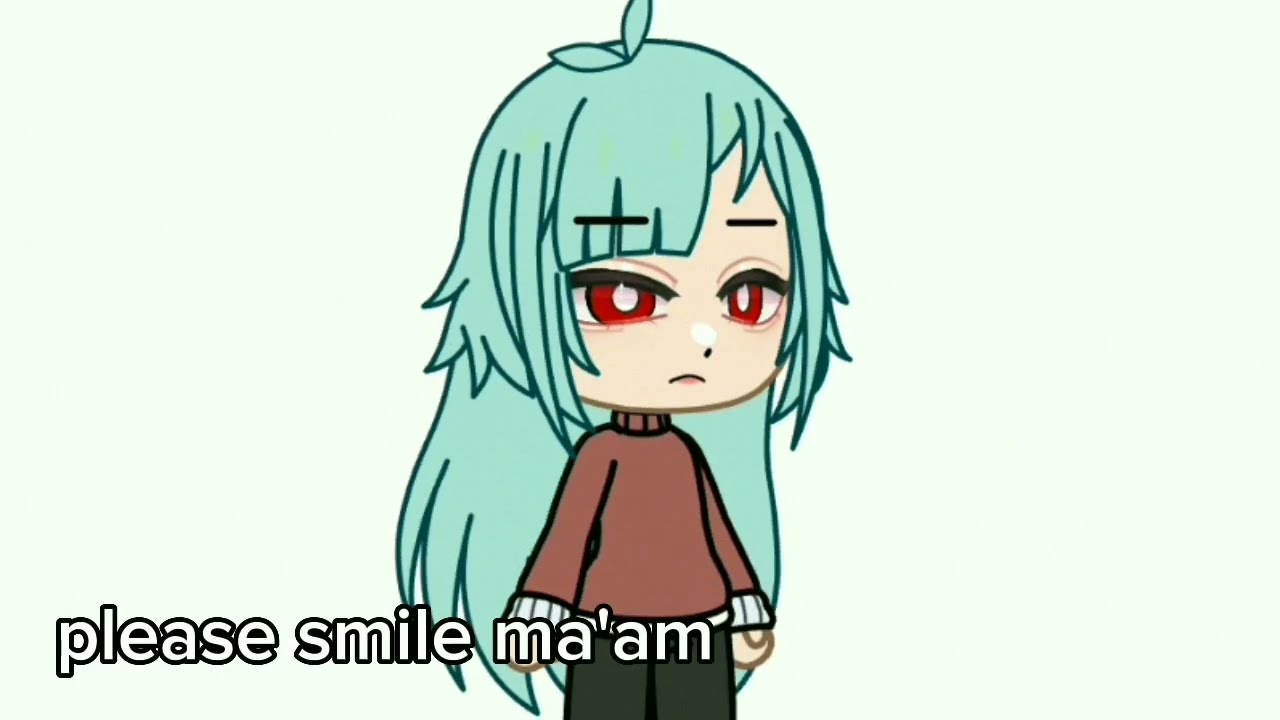The digital art piece features a centered anime-style young girl with striking long aquamarine hair cascading down to her legs. Her hair, full and vibrant, frames her face with bangs that partially cover her left eye, while the right side is neatly parted. She has a pale peach complexion accentuated by thick black eyebrows and prominent red eyes with large white pupils, giving her an expressive, almost somber look. Her outfit consists of a light brown turtleneck sweater adorned with white cufflinks and olive green pants. The background is a light green hue, complementing the color palette of the character. Positioned slightly to the left yet still central, she gazes forward with a frown, and at the bottom of the image, there is text that reads, “please smile ma'am,” adding a touch of narrative to her expression.